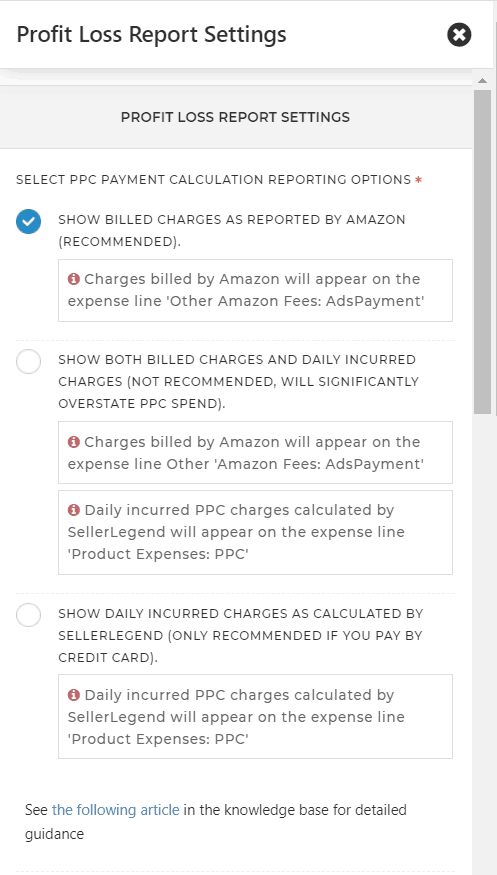In this screenshot, the interface displays various settings for a "Profit Loss Report." At the top, a white header reads "Profit Loss Report Settings." Below this, on a gray background within a box, the title "Profit Loss Report Setting" is shown again. Further down, against a white background, it says "Select PPC Payment Calculation Reporting Options."

Underneath, there is a blue circle with a white check mark next to the option that reads "Show billed charges as reported by Amazon (Recommended)." This is followed by a description in another box that states, "Charges billed by Amazon will appear on the expense lines. Other Amazon fees add payment."

Below that, there is another option: "Show both billed charges and daily incurred charges (Not recommended, will significantly overstate PPC spend)," with a circle to the left indicating its selection status. The final option is "Show daily incurred charges as calculated by Seller Legend (Only recommended if you pay by credit card)," also accompanied by a circle indicating its selection status.